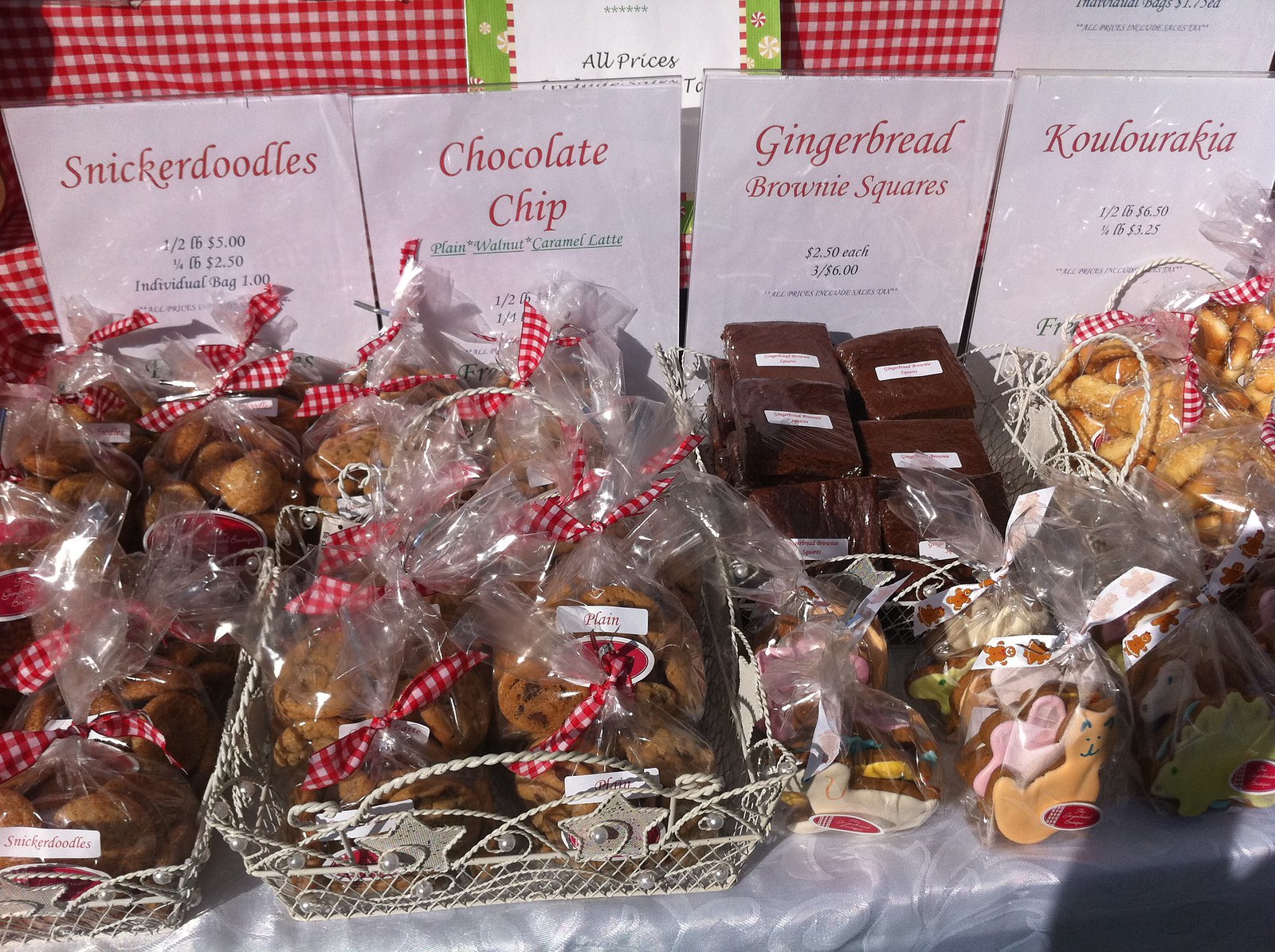This color photograph, rectangular in shape, captures a beautifully arranged bake sale display on a table covered with a shiny white, silky tablecloth. The table is adorned with various bags and packaged treats, each delicately wrapped in clear cellophane and tied with charming red and white gingham ribbons. Behind the array of baked goods, a series of white signs, held upright in plastic stand boards, clearly describe the items and their prices.

To the left, there is a sign for snickerdoodles, with prices listed as half a pound for $5, a quarter pound for $2.50, and $1 for an individual bag. In front of it, a wire basket holds neatly packed snickerdoodles, each bag tied off with the aforementioned ribbon. Moving to the right, there is another sign listing chocolate chip, plain, walnut, and caramel latte cookies. The basket below features these cookies, wrapped in the same charming manner, and the prices, though less visible, hint at a similar format.

Further to the right, a sign announces gingerbread brownie squares priced at $2.50 each or three for $6. These dark brown square treats are also elegantly wrapped in plastic with white labels. In front of this display, smaller plastic bags hold animal-shaped cookies, featuring a playful assortment that includes a yellow cat and a green dinosaur.

At the extreme right, there is a sign indicating kouroulakia, traditional Greek twisted cookies, priced at half a pound for $6.50 or a quarter pound for $3.25. These small brown twisted confections, bagged similarly to the others, are reminiscent of soft pretzels but distinctly different in appearance and texture. The entire setup, against a checkered white and red backdrop, exudes a delightful, inviting atmosphere typical of a well-organized bake sale.